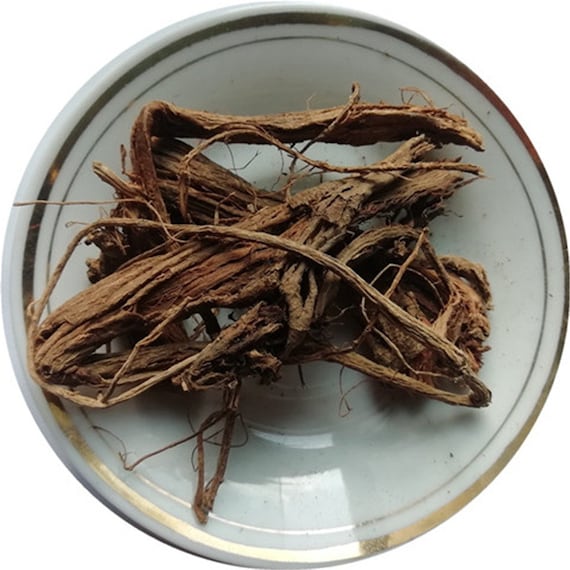This image shows a confusing but intricate scene of a brown, stringy material resembling roots or extracted plant stems, placed on a round white ceramic plate. The plate has a prominent gold-colored border that alternates between the outer and slightly inner rim as it circles around. The material itself, which appears brown and coarse with both grainy and wiry textures, is arranged with a notable horizontal piece on top and several thick and stringy pieces extending in various directions. Despite its unusual presentation suggesting nature or origins from the ground, the setup with this glossy plate, reflecting sunlight, implies it might be something one would consider for consumption. The light teal hue of the plate, though appearing almost cream, adds a subtle touch of elegance to this peculiar yet intriguing scene.